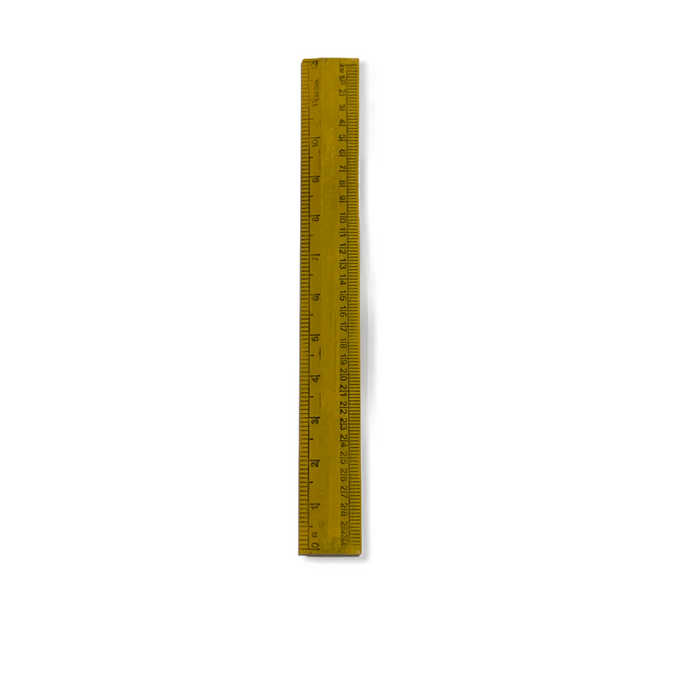This image showcases a well-worn, wooden ruler, laying flat on its side against a stark white background. The ruler, appearing slightly yellowish and dirty, features both inches and centimeters, with the inch markings on the left and centimeter markings on the right. Spanning up to 12 inches on one side, it has smaller, evenly spaced black markings for millimeters or centimeters on the other. The ruler's surface shows signs of heavy use, including faded markings, especially near the 11th inch, and black stains suggesting it hasn't been cleaned in a while. The lines and numbers are printed in black. A subtle shadow appears towards the right of the ruler, adding depth to its otherwise minimalistic setting.